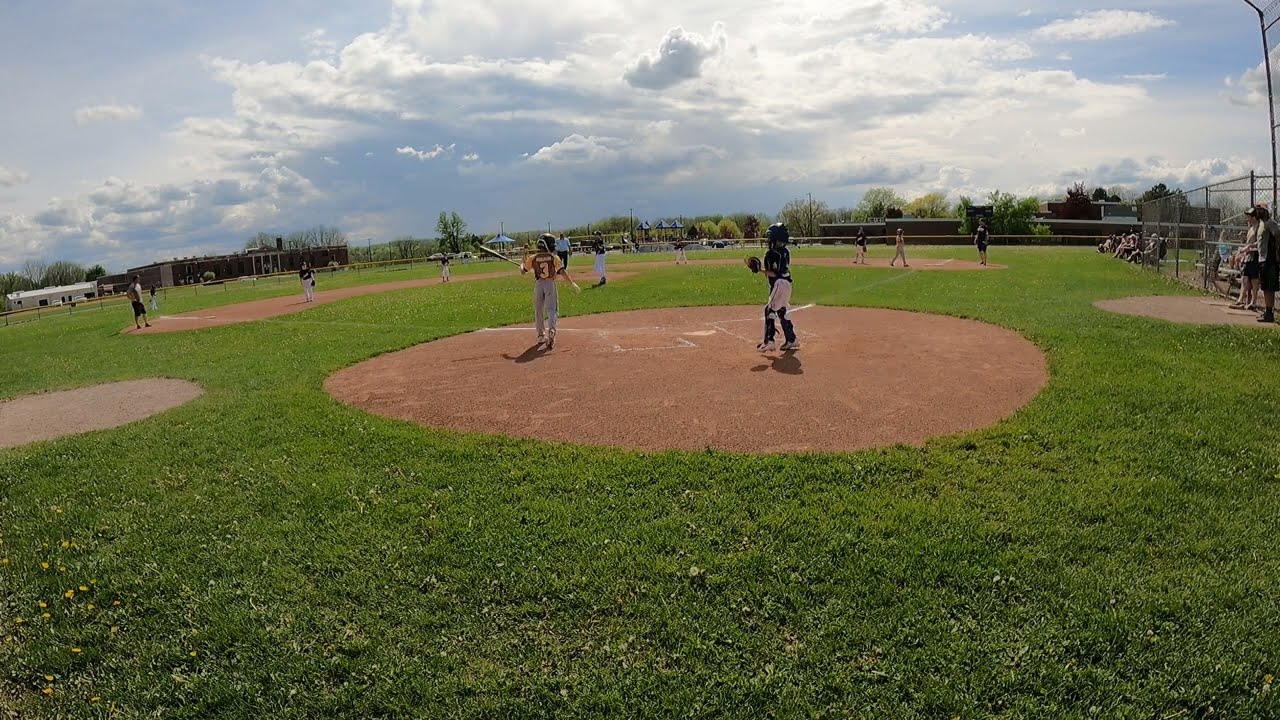The image captures an action-filled moment of a youth baseball game, likely a middle school or little league event, taken from behind home plate. The scene is set on a mostly grass field with prominent patches of brown dirt and clay, especially around the pitcher's mound and home plate. In the foreground, the catcher and the batter are poised for the next play, while the pitcher and infielders are positioned and focused on the game, their backs to the camera. The defending team, dressed in blue jerseys with white trousers, holds down the bases, with a coach standing near third base, possibly giving advice to runners.

To the right, the dugout is visible with coaches and a few spectators seated on bleachers beside the field, separated by a chain-link fence. In the background, beyond the field, a mix of green and light green hues from the trees stretches across the horizon under a mostly cloudy sky, which also reveals patches of blue and sunlight. Farther in the distance, there are buildings, one gray and another white, adding to the suburban setting of this lively outdoor event. The photo encapsulates the dynamic energy of the game, capturing the essence of a sunny yet partly cloudy day.